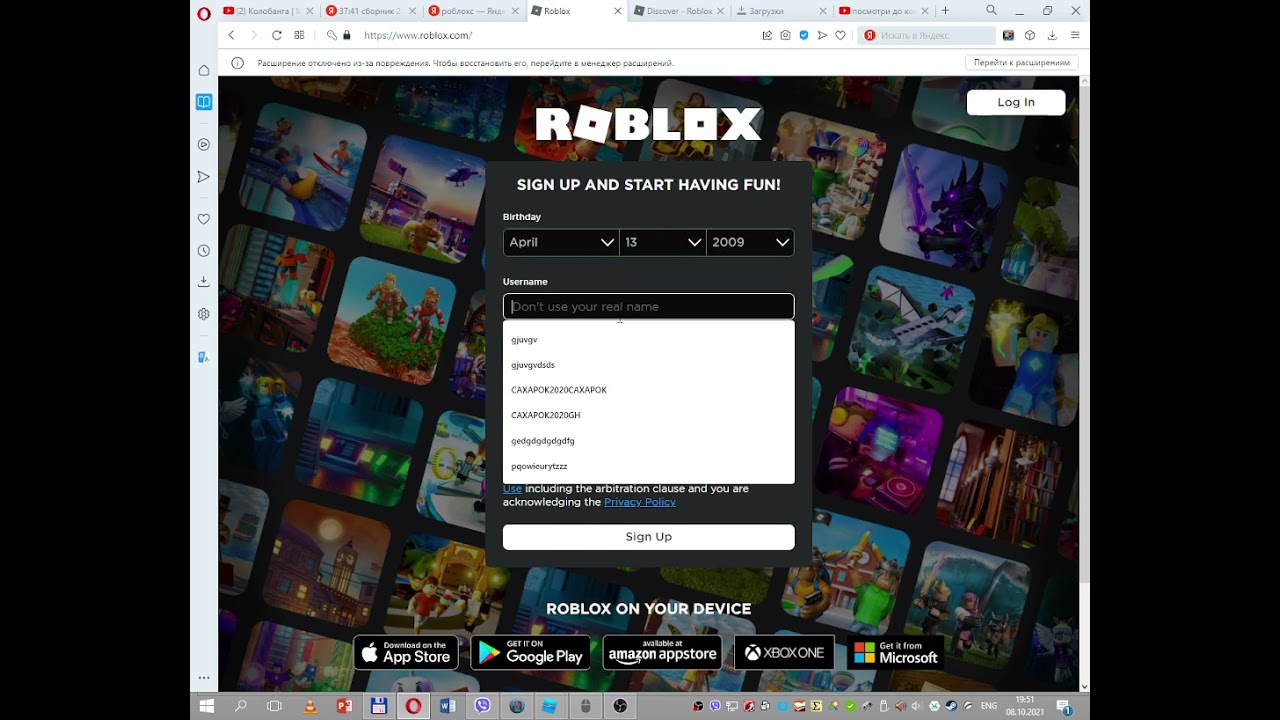The image depicts a computer screen displaying a web page related to Roblox, a popular gaming platform. The page prominently features the Roblox logo and a call-to-action message encouraging visitors to "Sign up and start having fun." The top section of the browser’s web bars contains text that is very small and difficult to read. 

In the background, there are various images representing different games available on Roblox, creating a dynamic and appealing visual. A drop-down menu can be seen on the page with numerous options, although the text is too small to decipher. 

Towards the bottom of the screen, a series of clickable boxes provide links to different platforms where Roblox is available. These include the Apple Store, Google Play, Amazon, the App Store, Xbox One, and Microsoft. Notably, the Microsoft box features the recognizable Microsoft logo, comprising four colored squares: red, green, blue, and yellow.

At the very bottom of the web page, there are numerous small icons, presumably links to various sections or features, though they are too tiny to identify specifically. The overall layout suggests a well-organized, user-friendly interface geared towards enhancing the gaming experience.